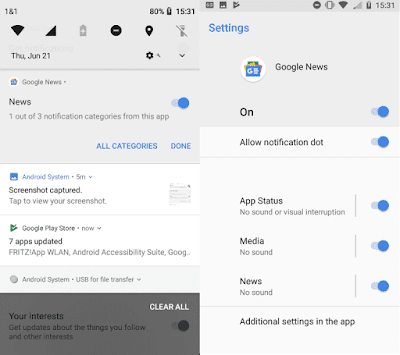A disorganized smartphone screen displays an array of notifications and interface elements. Key highlights include the "Do Not Disturb" feature being activated, with a location pin and an inactive torch light icon. The status bar shows the date as Thursday, June 21st and the time as 15:31, with signal strength at one bar and Wi-Fi fully connected. The Bluetooth settings are also visible. 

A gear icon suggests access to the settings menu, which, upon further inspection, reveals a Google News section labeled "News" with one out of three notification categories active. Various toggles for notification categories and an "All Categories" option are noted, alongside a “done” button.

Notifications indicate a screenshot capture prompt to view the screenshot and an update status from the Google Play Store, reporting that seven apps, including the Fritz app and WLan, have been updated. The Android system note mentions USB for file transfer functionality.

Additionally, a blurred image of another smartphone screen displays more icons, reinforcing the presence of a "Do Not Disturb" and vibration-activated status. This screen features settings for loud notifications, app status, media, and news, though everything appears very out of focus, rendering finer details unclear.